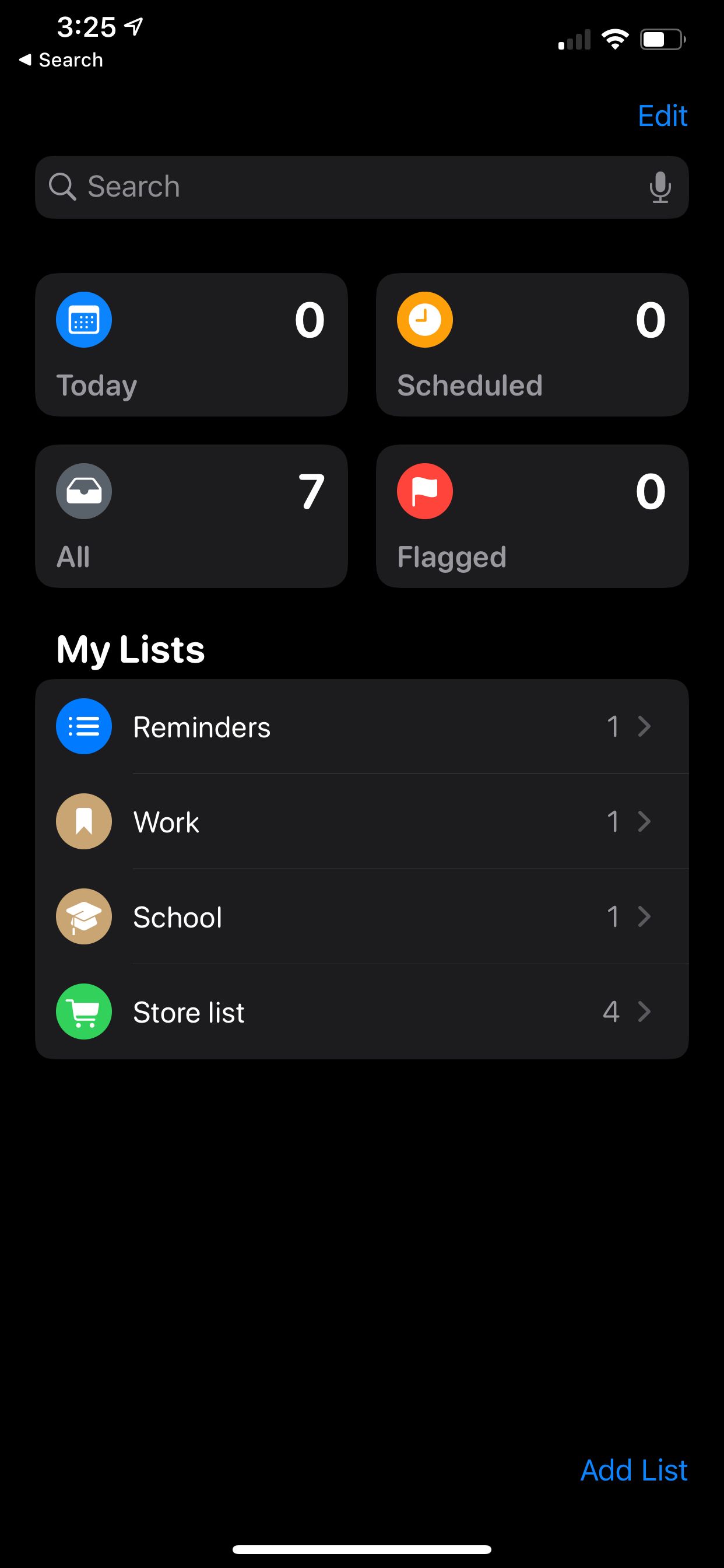This screenshot depicts an organized interface of a smartphone application with a distinctly dark theme. The background is black. At the top of the screen, the status bar displays the time "3:25," along with icons for signal strength, Wi-Fi connectivity, and battery level. Below the status bar, the word "Search" is centered, with the word "Edit" in blue text aligned to the right-hand side. 

A search bar resides beneath this header, featuring a magnifying glass icon and the word "Search" in white text, with a microphone icon on the right end of the bar.

The main content is organized into four distinct boxes arranged in a two-by-two grid. The first box in the upper left corner has a blue circle containing a calendar icon, labeled "Today," with the number "0" beneath it. The second box on the upper right features an orange circle with a clock icon, labeled "Schedule," also with the number "0." 

Directly below, on the left, a gray circular icon resembling a file drawer is labeled "All," with the number "7" underneath. The fourth box to the right showcases a red circle with a white flag icon labeled "Flagged," with the number "0."

Beneath these boxes, bold white text reads "My List," followed by categories listed as "Reminders," "Work," "School," and "Store List."